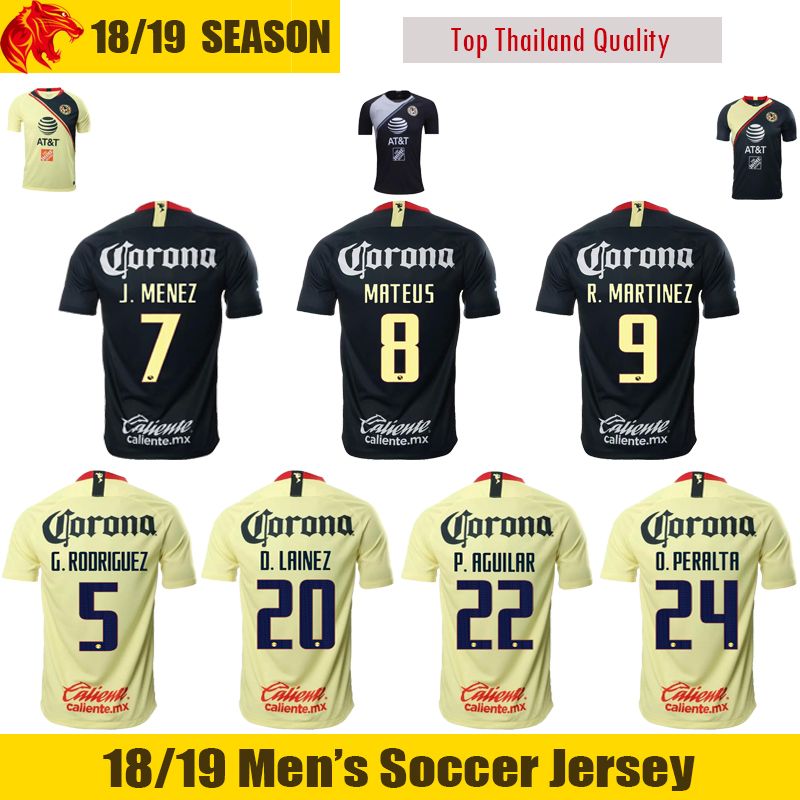The image showcases a diverse collection of soccer jerseys likely intended for a sales brochure or online catalog. The background is white, featuring several detailed pictures of jerseys. In the upper left corner, a gold rectangle with black text denotes the "18/19 season," accompanied by a side logo of a red tiger's mouth open. To the upper right, a gray rectangle with red text indicates "Top Thailand Quality." There are three rows of jerseys: 

- The top row presents the fronts of jerseys, including one white and two navy blue shirts, each emblazoned with the AT&T logo. 
- The middle row displays the backs of three navy blue jerseys, with player names Jay Menez (#7), Mateus (#8), and R Martinez (#9). Each bears the light blue "Corona" logo above their names, with names and numbers in white.
- The bottom row shows the backs of four white jerseys, also adorned with the "Corona" logo followed by player names G Rodriguez (#5), D Lanez (#20), P Aguilar (#22), and D Peralta (#24) in navy blue.

At the very bottom of the image, a yellow rectangle with black text concludes with "18-19 Men's Soccer Jersey."